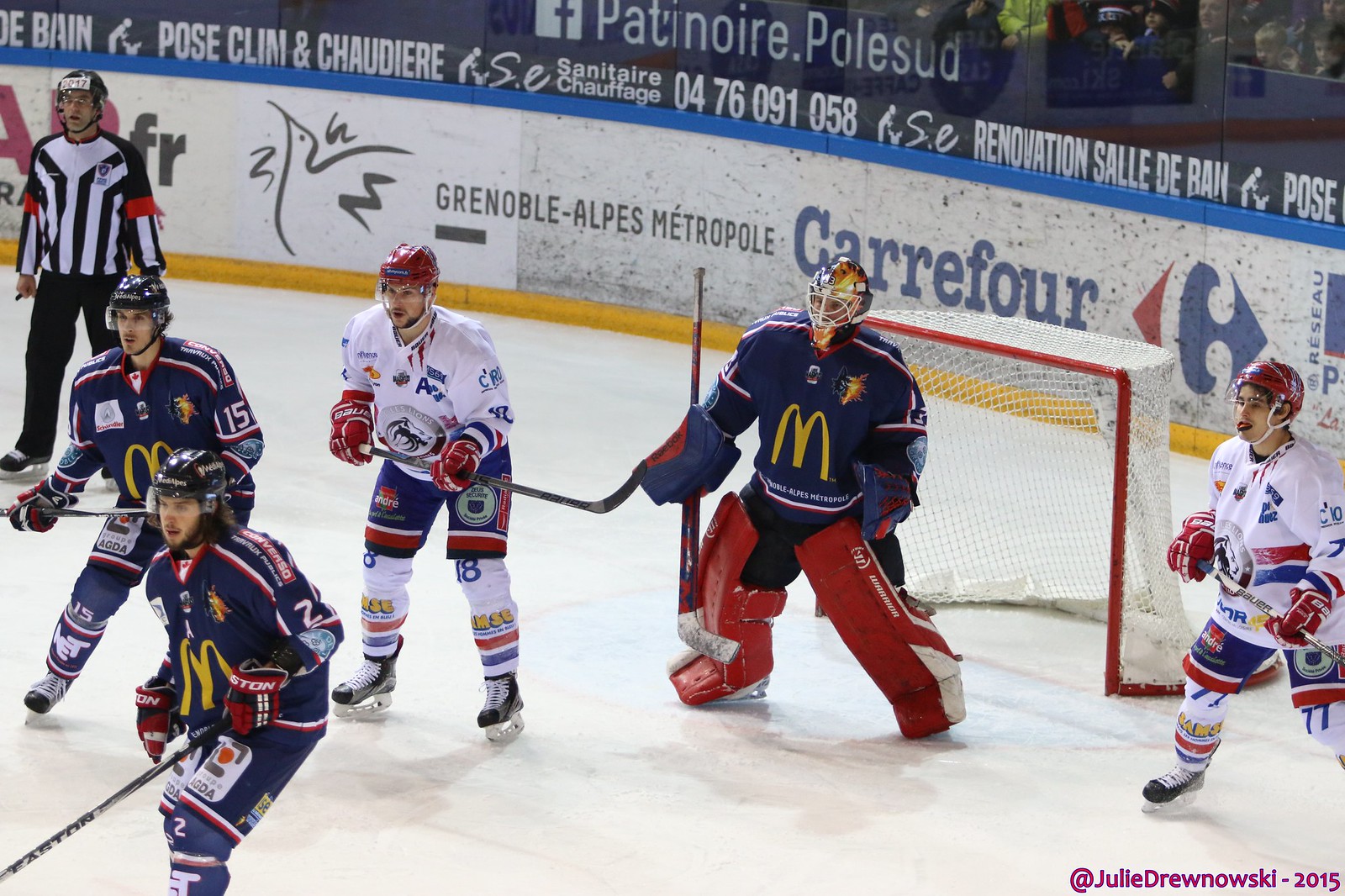The photograph captures an intense moment in a professional hockey game. The scene is centered on the goalie of the team in blue uniforms, prominently displaying a McDonald's emblem on their chests, likely indicating sponsorship. The blue team’s goalie is equipped with red leg guards, standing alert in front of the goal. Surrounding him are two of his teammates, also in blue, positioned to defend against the opposing team.

The opposing team, dressed in white jerseys adorned with blue and red accents, has two players on either side of the goal, creating a tense standoff. Above them, fans fill the stands behind the goal, adding to the charged atmosphere of the game. A referee is visible in the upper right corner of the image, identifiable by his official attire and red bands on his shirt sleeves.

The arena's edge is lined with various advertisements in a foreign language, suggesting an international location, possibly Canada. Advertisements spotted include "Chernobyl – Alps Metro Pole," "Cary 4," and ads for renovation services and student-oriented promotions. Notably, the bottom part of the image features a watermark or credit that reads "at Julie Dronowski – 2015."